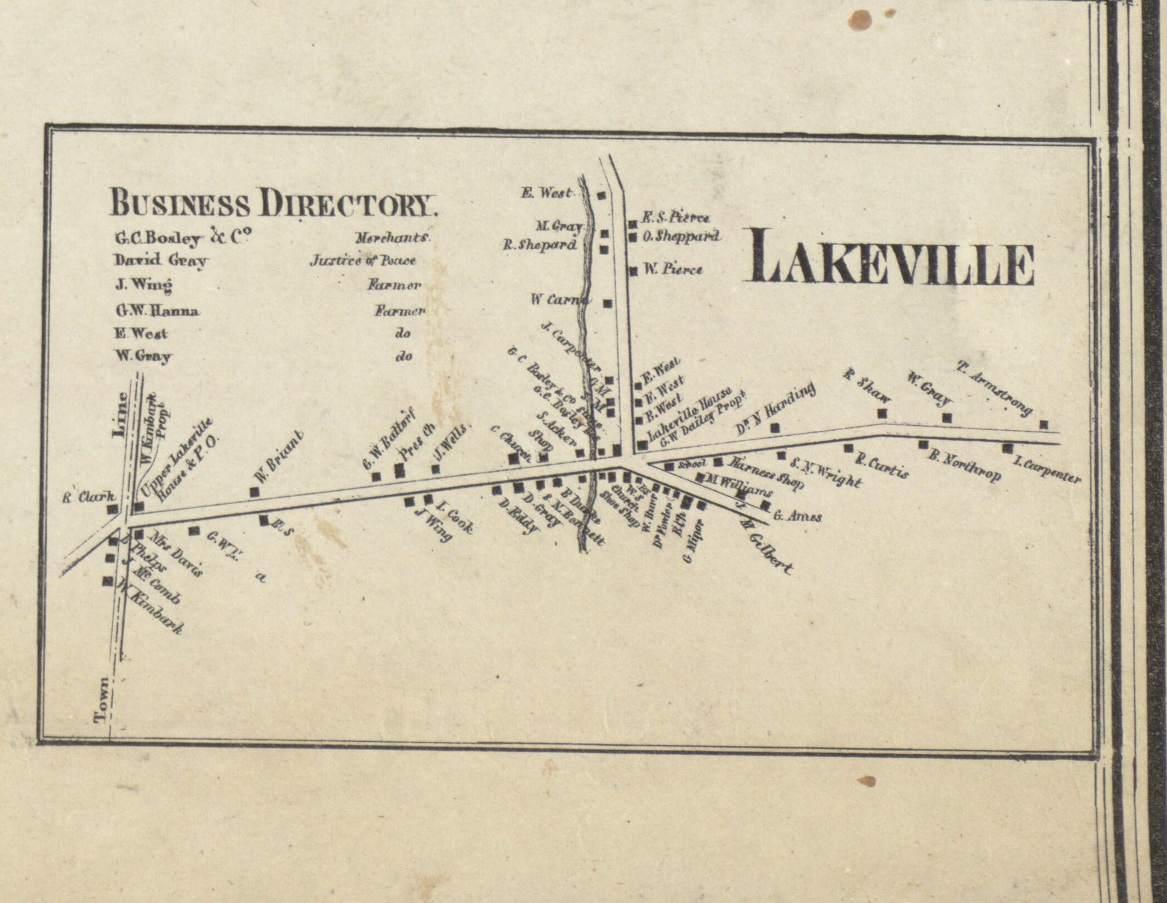The image depicts an old, yellowed piece of paper that appears to be a map or business directory. The paper has a tan background with a black border enclosing the map. In bold black text at the top left within a prominent black rectangle, it reads "BUSINESS DIRECTORY." Adjacent to this, on the top right corner of the page, the text "LAKEVILLE" is displayed in all caps. Below "Business Directory," several names are listed: G.C. Bosley, David Guillet, J. Wing, J.W. Hannah, E. West, and W. Gray. The map suggests a layout of streets and locations with additional names and descriptions such as merchants, justice of peace, and farmers, though some of these details are not legible. The directory includes various names and appears to point out specific buildings or homes, like the Upper Lakeville House and Post Office and mentions of significant figures such as R. Clark, W. Kimbark, J. McComb, and others, indicating the residences or businesses associated with these individuals.